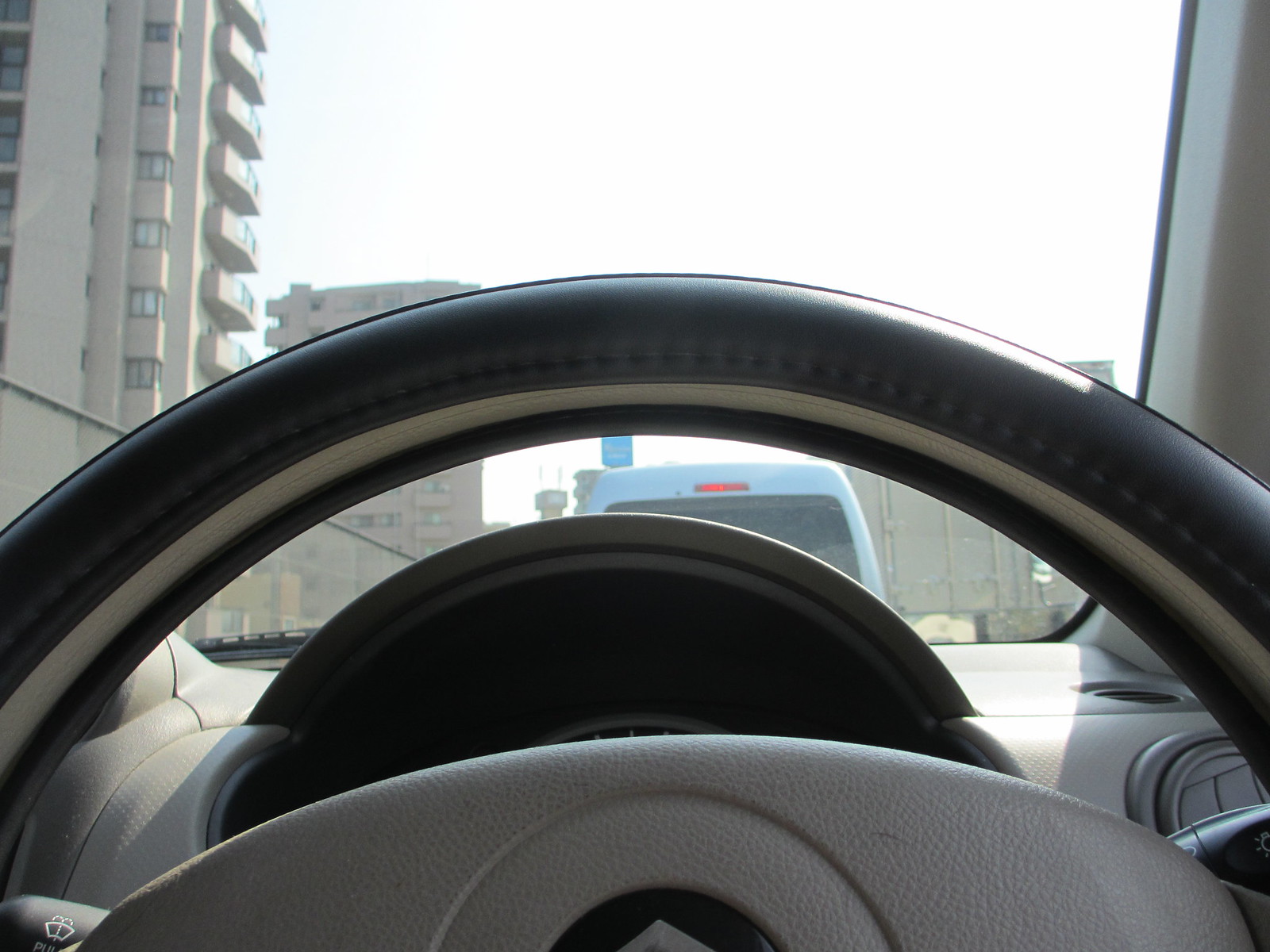The photograph, taken from the interior of a right-hand drive European car, captures a detailed view from the driver's perspective. The focal point is the steering wheel, prominently displayed in the foreground, with its black leather cover and a gray center possibly featuring an unclear logo. The dashboard is largely obscured, but the arced design and the presence of air conditioning vents are noticeable.

Beyond the steering wheel, the viewer's gaze is drawn through the windshield to an overcast sky, rendered in a hazy white. In the upper left corner, a multi-story tan apartment building rises, while just below, the roof of a white van is visible. The right edge of the image reveals a tan pillar supporting the windshield, reinforcing the impression of sitting inside a compact vehicle. The interior's color palette consists mainly of tans and grays, contrasting the black leather steering wheel cover. Overall, the image captures a mundane yet intimate moment inside a car, set against an urban backdrop.